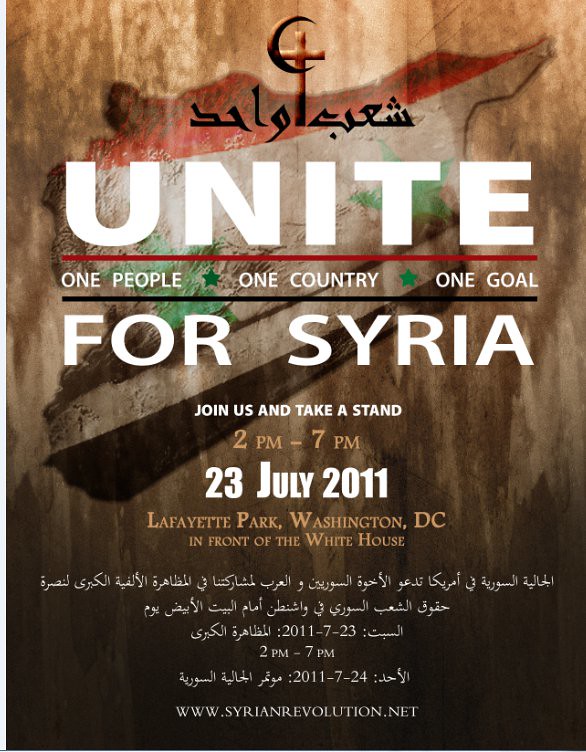The image is a promotional poster for an event supporting Syria. At the top, there is a symbol combining a Christian cross and an Islamic crescent moon, accompanied by Middle Eastern script. In large, bold white letters, the word "UNITE" is prominently displayed. Below that, separated by a red line, is the phrase "one people, one country, one goal," with green stars serving as bullet points. The text "FOR SYRIA" follows underneath, inviting readers to "join us and take a stand" from 2 p.m. to 7 p.m. on July 23rd, 2011, at Lafayette Park in Washington D.C., right in front of the White House. The background features the Syrian flag, shaped to resemble the country, and stained with dark liquid artifacts. The poster also includes a website at the bottom: www.syrianrevolution.net.